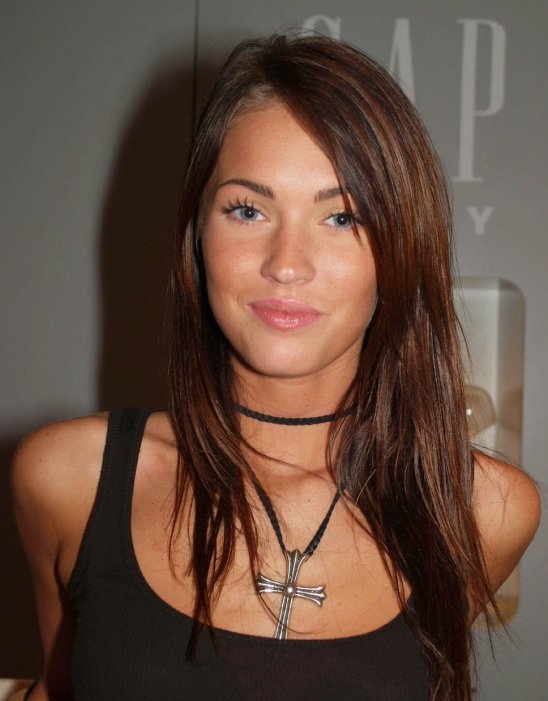This color photograph showcases a young Megan Fox, the American actress, posing in front of a GAP branded backdrop. She stands facing forward with her long brown hair flowing over her shoulders, partially covering her black tank top. Her arms are positioned behind her back, giving the appearance that she is slightly leaning backward. Megan's expression is a closed-mouth smile, enhanced by her pink lipstick. Around her neck, she wears a distinctive black rope or leather necklace with a large silver cross pendant resting on her chest. The background features a gray wall with partial text, identified as “GAP,” and possibly other symbols or letters obscured by her presence. The image captures only her head, shoulders, and the upper half of her chest, highlighting her bright eyes, thin nose, and overall poised demeanor.